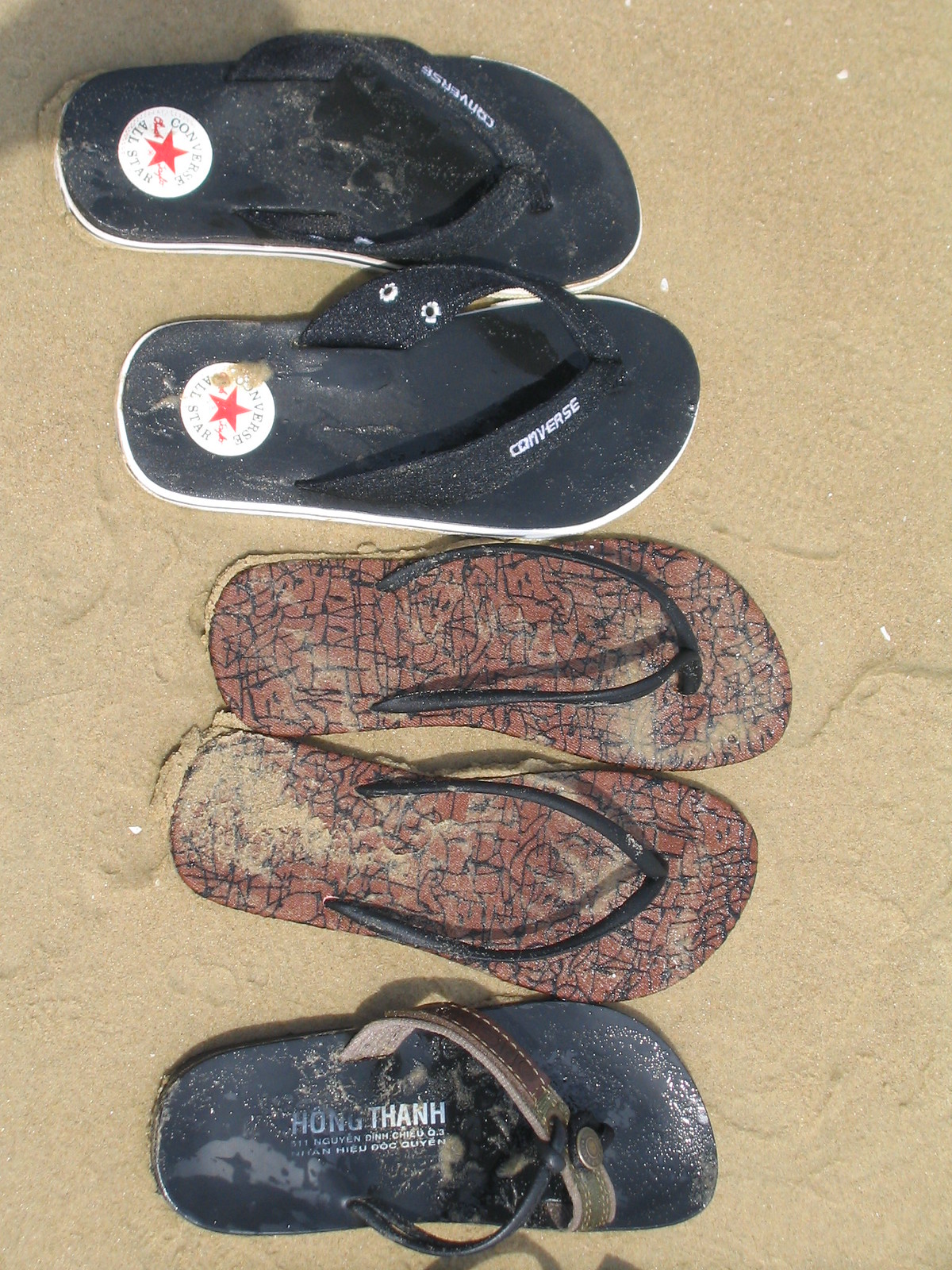This close-up photograph captures an assortment of beach footwear lying on wet sand, taken from an overhead perspective. The image prominently features two pairs and one loose sandal. At the top, there’s a pair of black Converse sandals with the distinct "Converse All-Star" logo on the heel and white edging around the sole. The second pair, positioned below the Converse, features a thin, black thong strap and a dark reddish-brown cork sole speckled with black highlights. Finally, a single sandal appears at the bottom of the frame, recognizable by its black base, leather strap, and partially legible "Hong Thanh" branding. The sandals rest on sand that displays traces of both dry and wet textures, adding to the beach ambiance of the scene.